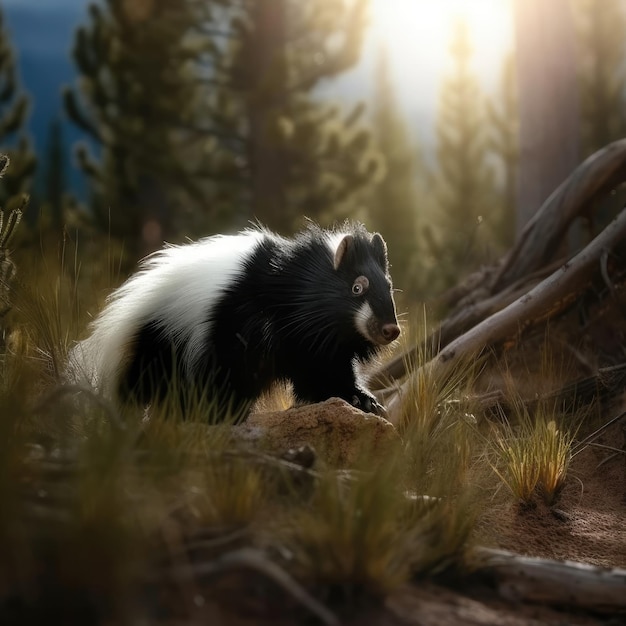The close-up image, presumably a photograph or hyper-realistic AI-generated picture, depicts a skunk in a natural setting. The skunk, primarily black with white markings beneath its jaw and down its back, is positioned slightly to the left and at a three-quarters angle, peering towards the viewer with one eye and its ears perked up. Its front left paw rests atop a small mound of dirt, surrounded by tufts of grass and scattered branches. The scene includes a mix of fallen trees or roots and standing palm trees on the left, along with a larger tree's roots visible on the right. In the blurred background, the sun is flaring just out of the frame, creating a bright spot at the photo's top. Pine trees are faintly visible amidst the sunlight. The skunk’s positioning and the natural elements, such as rocks and a few emerging plants, add to the serene, pastoral atmosphere of the scene.